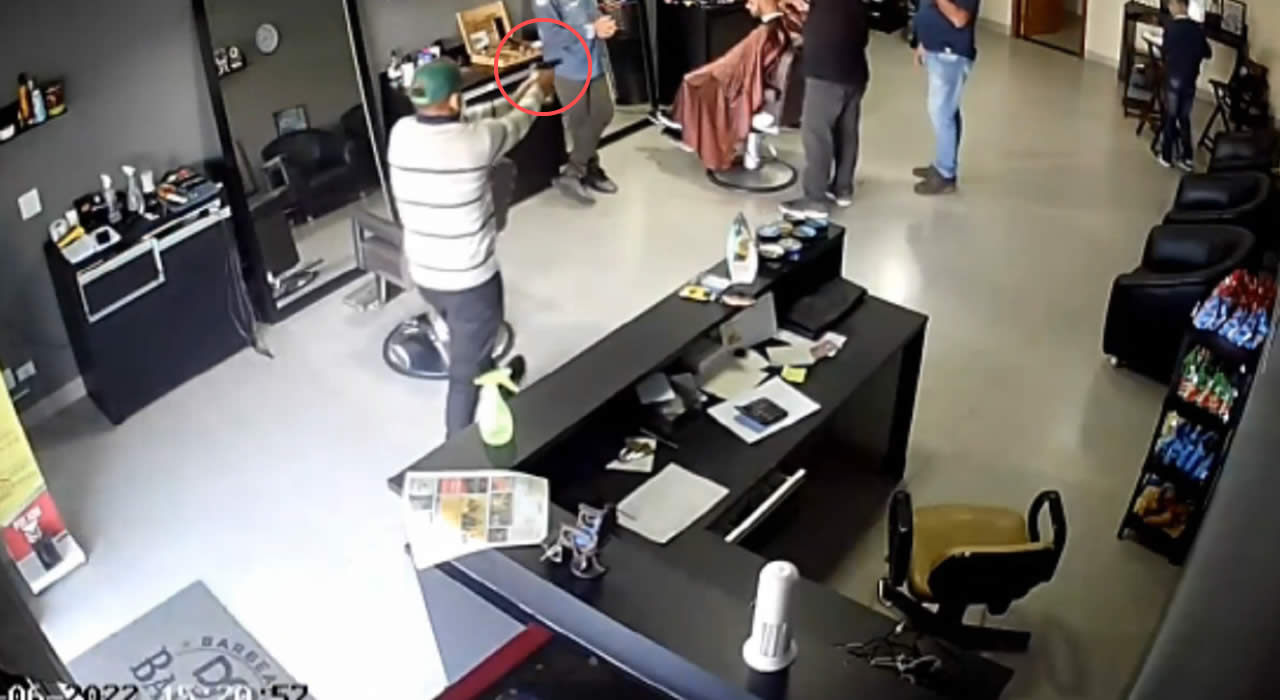The image depicts a tense scene inside a barbershop. There are seven patrons and one barber present. One patron sits in the chair getting a haircut from the barber. Another man stands behind them, while a third man leans against the counter. Several additional patrons are seated in waiting chairs. The barbershop features a chip rack, full-length mirrors with various barber products atop dressers, and a front desk with an office chair behind it. The floors are white tile, and the walls are gray. A man has just entered the barbershop, wearing a green baseball cap, a white shirt with black stripes, and gray slacks. He is aiming a handgun, which is circled in red, though none of the patrons or the barber seem to have noticed or reacted yet. The timestamp on the image reads June 2022, 15:20:57.